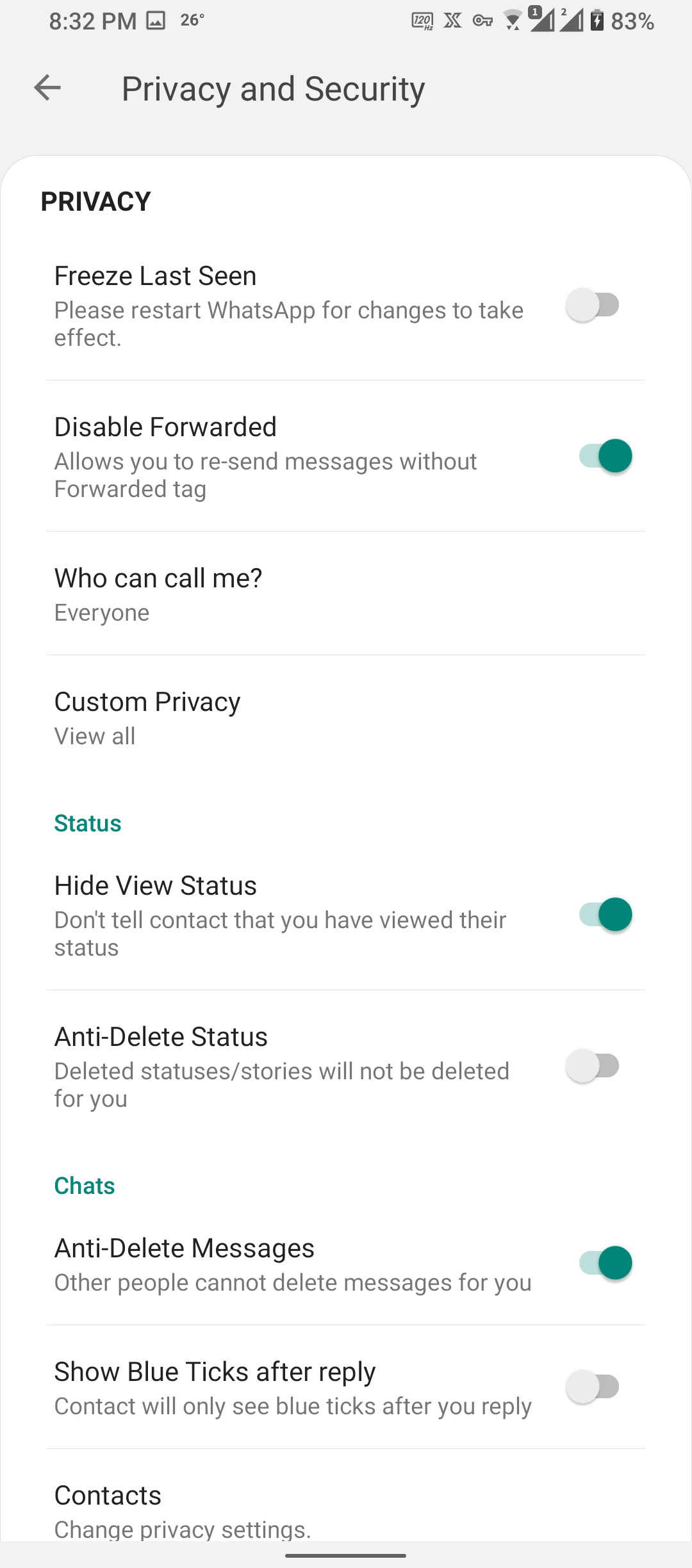**Descriptive Caption:**

This image is a screenshot of a smartphone display showing the time at 8:32 PM and the temperature at 26 degrees. The background is grey. At the top of the screen, icons indicate a strong Wi-Fi connection and a battery life of 83%. 

Below this, the screen details several privacy and security settings within an app, likely WhatsApp:

1. **Privacy and Security Section:**
   - **Freeze Last Seen:** This setting is currently off (displayed in grey). It informs the user to restart WhatsApp for changes to take effect.
   - **Disable Forwarded Tag:** This feature is on (displayed in green), allowing the user to forward messages without the forwarded tag.
   - **Who Can Call Me:** This setting is configured to allow calls from everyone.
   - **Custom Privacy:** An option to view all custom privacy settings.

2. **Status Section:**
   - **Hide View Status:** This feature is on (displayed in green), which means the user’s contacts will not be notified when their status is viewed.
   - **Anti-delete Status:** This setting is off (displayed in grey), meaning deleted statuses or stories will still be removed for the user.

3. **Chats Section:**
   - **Anti-delete Messages:** This feature is on (displayed in green), preventing other people from deleting messages for the user.
   - **Show Blue Ticks After Reply:** This setting is off (displayed in grey), which means contact will only see blue ticks indicating a message has been read after the user responds.

4. **Contacts Section:**
   - An option labeled "Change Privacy Settings."

The section contains a mix of black and grey text on a white background, with the active settings highlighted in green. A thin grey line and a grey box line separate these sections.

This detailed visual provides a comprehensive overview of various privacy settings within the app, helping the user manage their privacy according to their preferences.